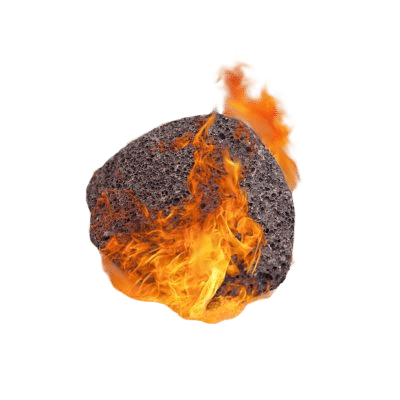This image depicts a small, rounded piece of coal or possibly a charcoal or lava rock, engulfed in vibrant flames. The rock is distinctly dark gray to black in color, with varying textures including grayish-white areas and numerous holes and air pockets scattered across its surface. The flames are rendered in vivid hues of yellow, orange, and dark orange, curving up both in front of and behind the rock, with a higher concentration of vibrant colors at the base. The entire scene is set against a stark white background, emphasizing the fiery spectacle and the detailed, porous surface of the coal. The flames at the back appear slightly blurred, adding a sense of depth, while the flames at the front are more defined. The overall impression is that this image, seemingly digitally or software created, isolates the burning rock against the clean background, leaving no other elements to distract from the intense display of fire and form.